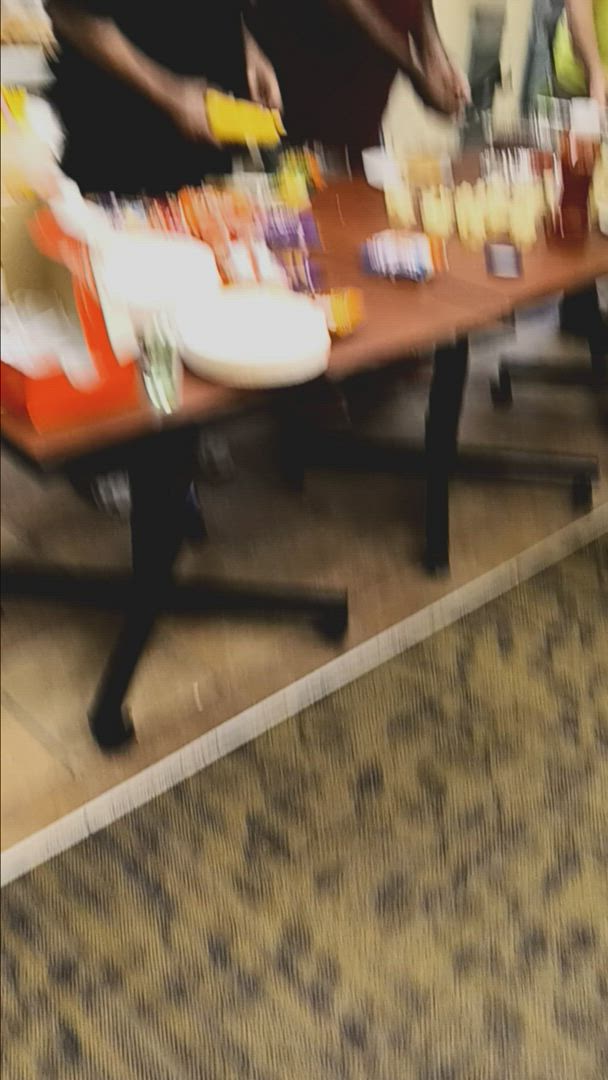In this long, vertical portrait photograph, a palpable sense of motion permeates the scene, which is defined by its blurry, almost ethereal quality. The focal point is a large wooden table with sturdy black legs, set against a stone or vinyl floor. Adjacent to the table lies a gold-colored carpet adorned with intricate black patterns, adding a touch of opulence to the setting. Atop the table are numerous party food items and disposable paper plates, though their features are lost within the motion blur that obscures specific details. Surrounding the table, three figures are captured in motion, their outlines indistinct and ghostly due to the blur, which transforms them into vibrant streaks of color. The image exudes a dynamic energy, evoking a sense of activity and festivity in an otherwise fleeting moment.